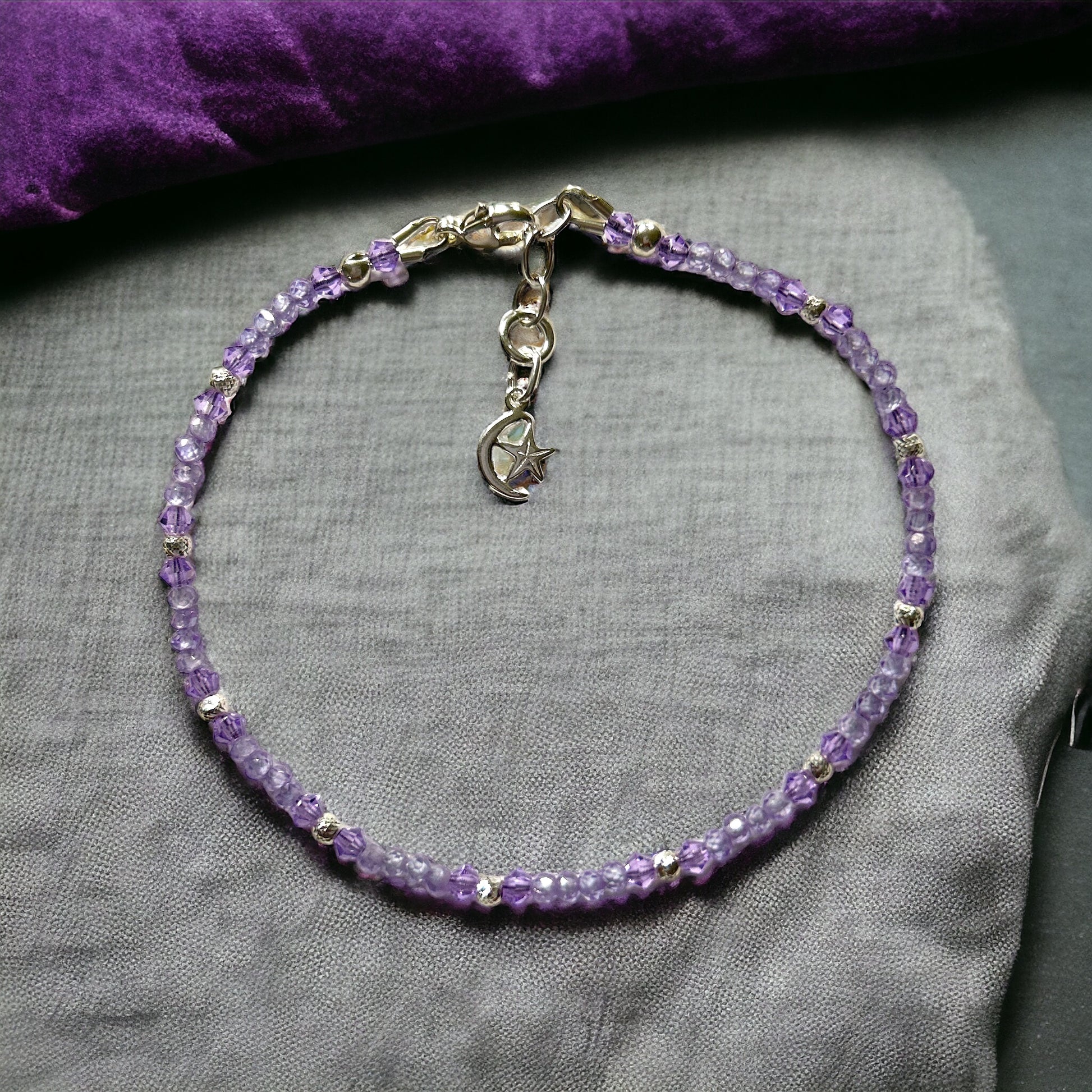The image showcases a circular necklace made predominantly of purple beads interspersed with silver or metal gray beads, creating a repeating pattern of about eight purple beads followed by one silver bead. The necklace is neatly clasped into a circle and is laid out on a slightly weathered gray cloth with a hint of a purple cloth or pillow in the background. Dangling from the necklace is a charming pendant featuring a crescent moon with a star nestled in its curve, both crafted from silver. This elegant piece of jewelry combines the serene charm of lavender hues with the timeless beauty of silver accents, making it a striking necklace.